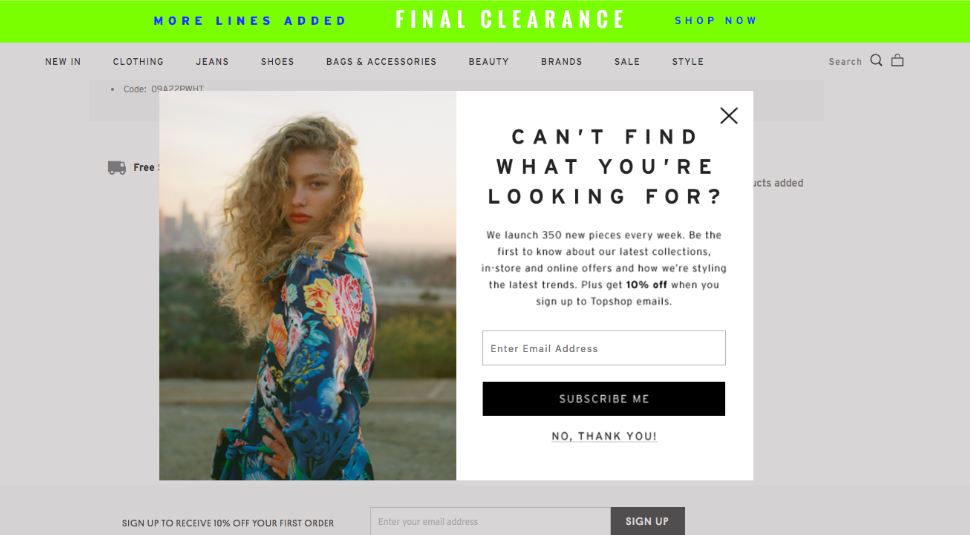The image depicts a promotional page from a clothing retail website, highlighting a clearance sale. The top banner of the webpage is adorned with a white and green message announcing "More Lines Added" and "Final Clearance," alongside a "Shop Now" call-to-action. Dominating the center of the page is a prominent pop-up designed like a postcard, which features an enticing offer: "Can't find what you're looking for? We launch 350 new pieces every week. Be the first to know about our latest collections, in-store and online offers, and how we're styling the latest trends. Plus, get 10% off when you sign up to Top Shop emails." Users are prompted to enter their email address and click "Subscribe Me." Alternatively, they can dismiss the pop-up by selecting "No Thank You" or clicking the X at the top corner.

Once the pop-up is dismissed, users are presented with various navigation options including "New In," "Clothing," "Jeans," "Shoes," "Bags and Accessories," "Beauty," "Brands," "Sale," and "Style." Peeking out from behind the pop-up is a sign featuring a small truck icon, likely indicating a free shipping offer, though the specifics may depend on a minimum purchase amount. Finally, the bottom of the page reiterates the 10% discount offer for new subscribers who provide their email addresses.